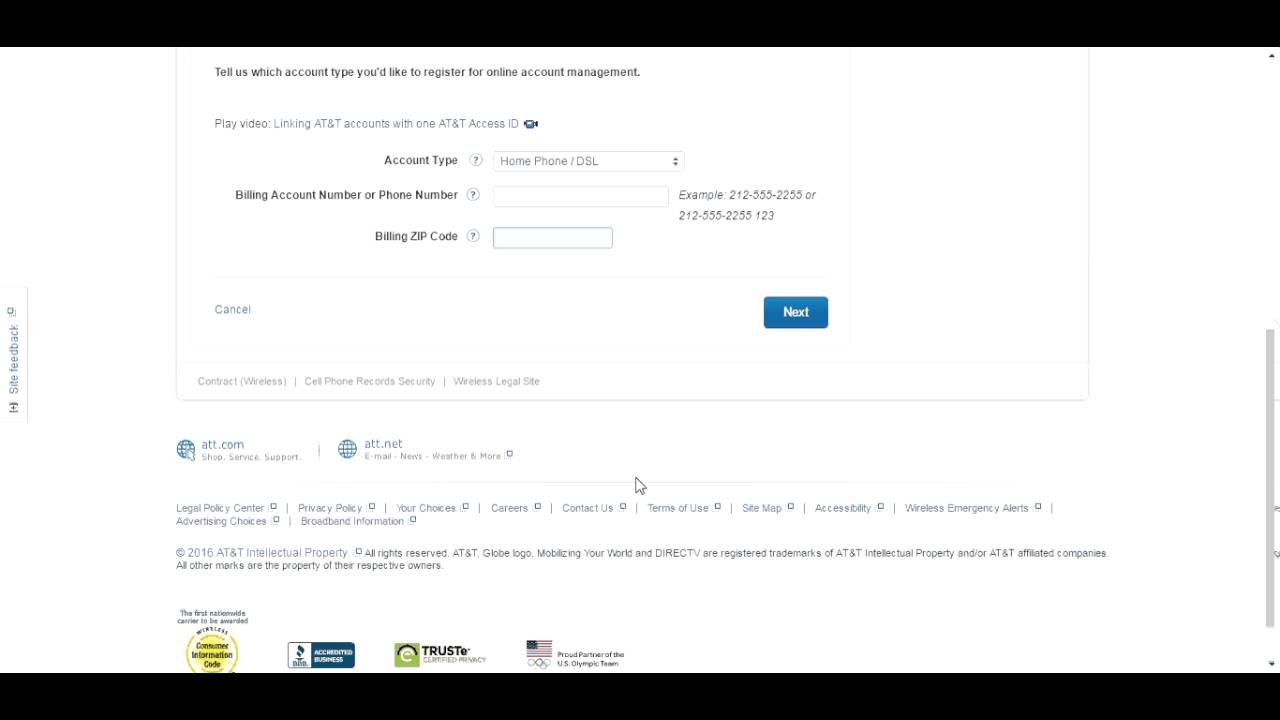This screenshot captures the final stage of an online purchasing process. The top portion of the website is partially cut off, obscuring the company logo. The webpage prompts the user to enter account details, which could be retrieved from their phone, along with a billing phone number or account number and the corresponding billing zip code, ensuring secure access to their phone records. 

A prominent "Next" button, displayed in a blue box with blue font, is visible, guiding the user to proceed. Additional information is listed below, including links to accessibility options, terms of use, and contact information for customer support.

At the bottom of the screen, several endorsements and certifications are displayed. The website is a proud partner of the US Olympic Team, highlighting a trust certification, and an accredited business badge. A Consumer Information Code award is also visible, signifying recognition for industry standards. Notably, the site claims to be the first nationwide carrier to receive this award, suggesting that it may belong to a delivery service provider.